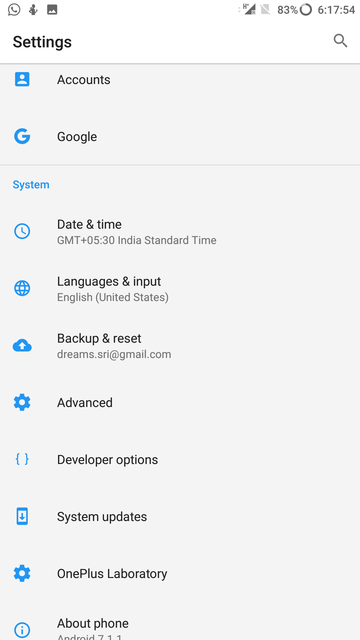This image is a screenshot of a smartphone's settings menu. At the top of the screen, indicators display the battery percentage and time. Below this, the word "Settings" is displayed in black text next to a small circular magnifying glass icon for search functionality.

The settings menu is divided into various sections:

1. **Accounts**:
   - A "Google" option marked by a blue "G" icon.
  
2. **System**:
   - **Date & Time**: A clock icon accompanies the text "Date & Time", showing the timezone as GMT+05:30 India Standard Time.
   - **Languages & Input**: Next to a globe icon, it indicates "Languages & Input" with the primary language set to English (United States).
   - **Backup & Reset**: A cloud icon with an upward arrow represents the "Backup & Reset" option, which includes an email address: dreams.sri@gmail.com.

3. **Advanced**:
   - A blue gear icon leads to "Advanced" settings.
   - "Developer Options" are enclosed in double parentheses. 

4. **System Update**:
   - This section features a blue smartphone icon with a downward arrow, marked as "System Update".

5. **OnePlus Laboratory**:
   - Another gear icon signifies the "OnePlus Laboratory".
  
6. **About Phone**:
   - A circular blue icon with an "i" in the center indicates the "About Phone" section, which shows the Android version as 7.1.1.

This comprehensive and organized layout offers a clear overview of the smartphone's settings and system information.